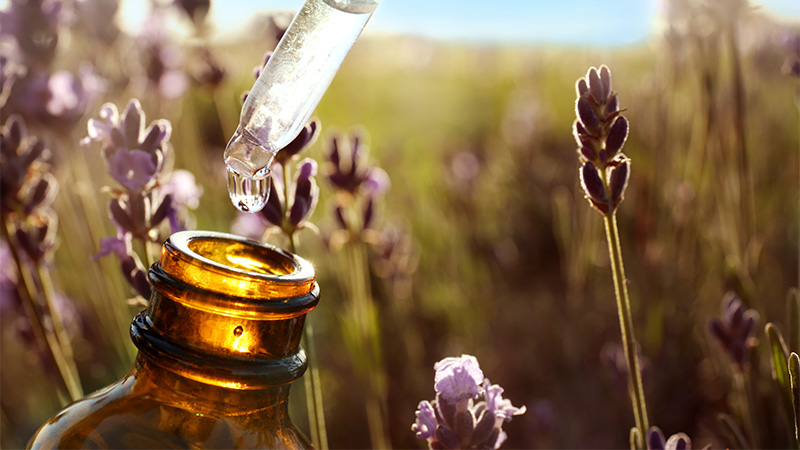This outdoor photograph taken on a sunny day showcases a close-up of a brown or amber-tinted glass bottle positioned in the lower left corner. Extending from the middle left side is an eyedropper, poised with a thick, translucent clear liquid droplet at its tip, ready to fall into the bottle’s open neck. The backdrop features a field of tall purple flowers with long stems, likely lavender, bathed in daylight and reflecting sunlight off both the bottle and the dropper. The flowers nearest the bottle are in focus, while the rest blend into a blur against a sliver of clear blue sky. The clear focus on the amber bottle and the dropper emphasizes the delicate action of the droplet about to descend.